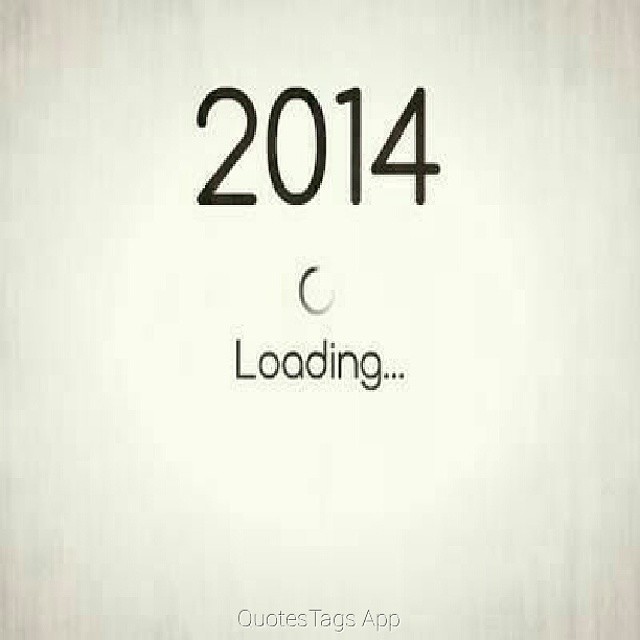In the image, there is a large light gray rectangle with a slightly darker gray gradient towards the corners, accented with streaks. At the center top of the rectangle, in heavy font, the year "2014" is prominently displayed in black and appears pixelated. Directly below it, there's a partially completed circle or a "C" shape facing the upper right, transitioning from dark black at the top to a lighter gray towards the bottom. This shape gives the impression of rotating or spinning. Underneath this shape, the word "loading" is written with a capital 'L' followed by lowercase letters and ending with three dots ("loading..."). At the very bottom of the image, in a subtle etched-like gray font, are the words "Quotes Tags App," each word starting with a capital letter. The overall design suggests a minimalist style, with essential elements centered and highlighted against a simplistic background.